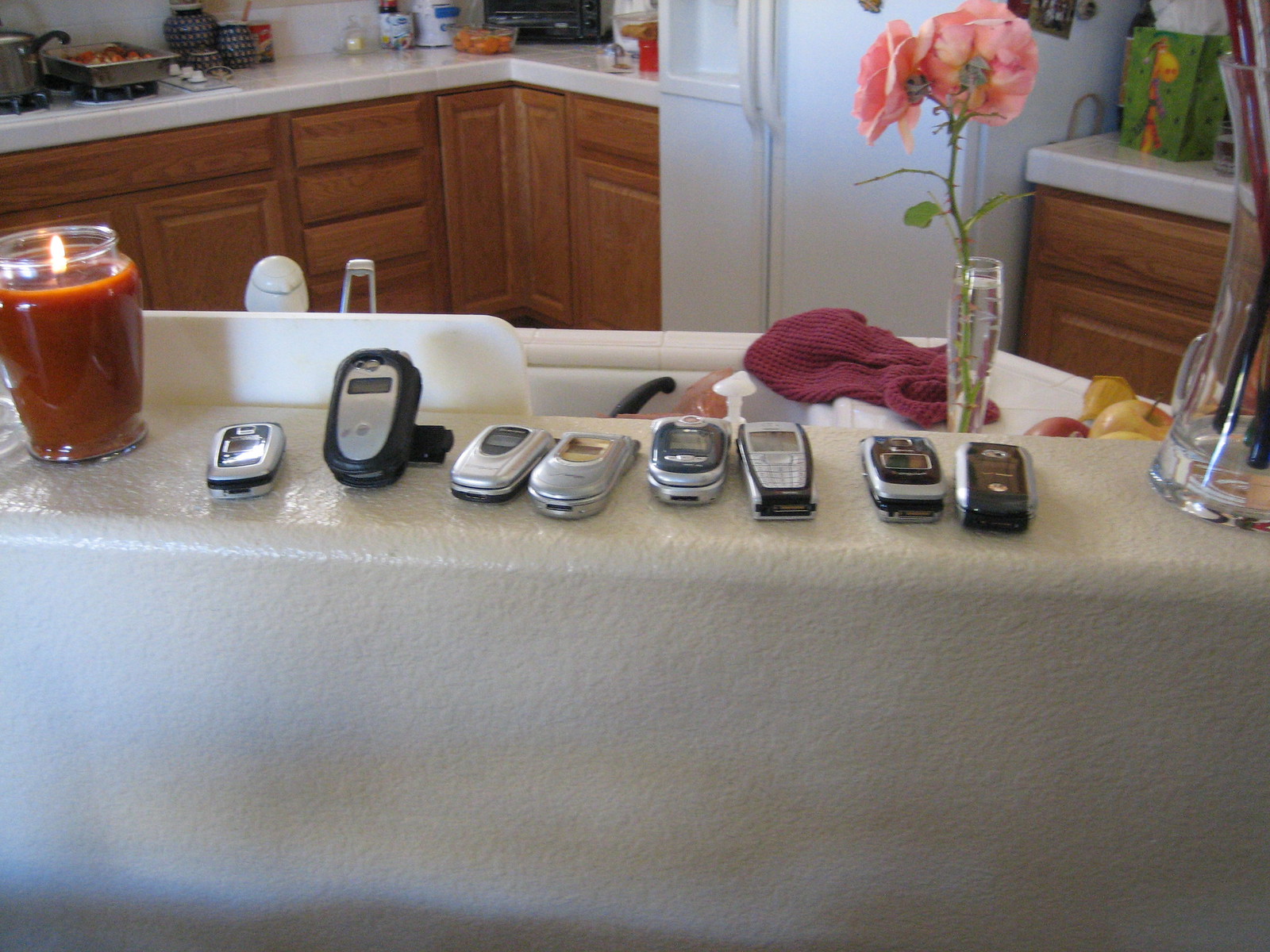In this brightly lit kitchen, a rectangular photo captures a nostalgic scene featuring eight flip phones, displaying a variety of gray and black hues, neatly lined up on a narrow countertop with a white sink. The countertop is adorned with a glass vase holding two vibrant pink flowers to the right of the sink and a lit candle in a dark brown, clear glass jar to the left. The kitchen background reveals brown cabinetry along the back and right walls, anchored by a white side-by-side refrigerator. Additional items, such as a burgundy dish towel, fruit, a black stainless steel pot, and a pan atop the left-side stovetop, contribute to the homely, lived-in atmosphere. The image hints at a family gathering, possibly reflecting a rule to place phones aside during meals to encourage conversation and face-to-face interaction.